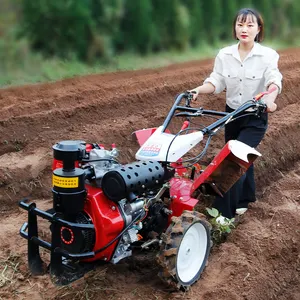The square image captures an outdoor scene where an Asian woman with shoulder-length hair is actively working in a farm field. She is dressed in a white button-up shirt with three-quarter sleeves rolled up, black pants, and white shoes. Positioned in the top right corner, she is maneuvering a robust red and black electric tiller machine across the soil. The tiller has prominent features including large black tires with white rims, a sturdy front bumper, and side chutes. The machine is angled towards the bottom left corner of the image, revealing its heavy-duty design aimed at plowing fields. The background further emphasizes the agricultural setting, with the bottom two-thirds showcasing evenly tilled soil and the top third adorned with lush green bushes and grass, highlighting the verdant environment.